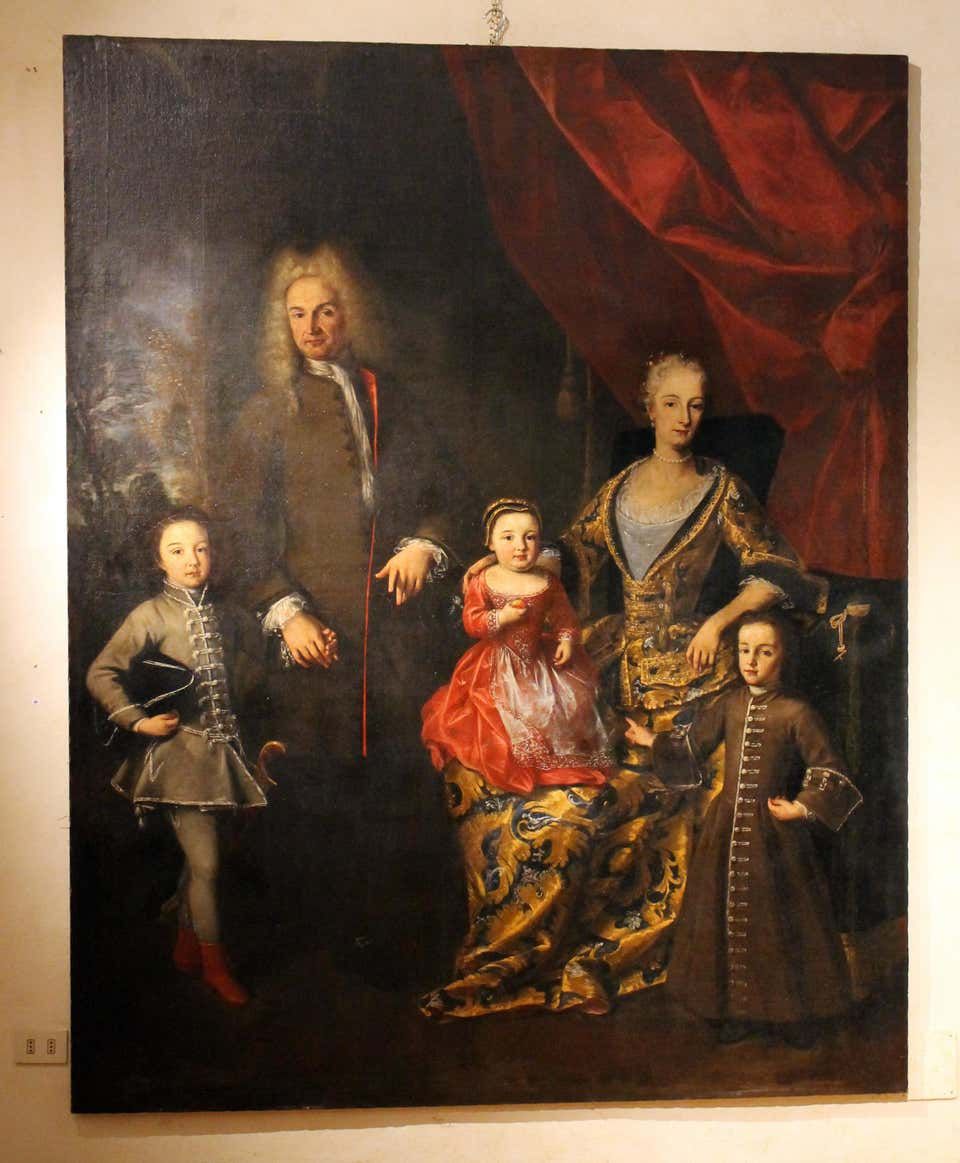This image is a detailed oil painting mounted on a white wall, featuring a family of five from what appears to be the Victorian era, rendered on a flat canvas with a small silver chain hook at the top for hanging. The family members are dressed in old-fashioned attire. To the left is a young boy, clad in a grey tunic with tight grey pants, red boots, and a grey coat, holding a black tricorn hat with white piping in the crook of his arm. He holds the hand of an older man who is adorned in a grey coat, a white scarf, and a traditional white wig. The man's coat sometimes appears to have red trim, but grey is the predominantly noted color. Seated next to them is a woman in a long, elaborate gold and black dress, cradling a small child dressed in a red dress on her lap. Standing to the woman's right is another young girl in a brown dress, possibly the second oldest in the family. The background of the painting features a dark tone with red drapery on the upper right side, adding depth and a rich atmosphere to the scene.